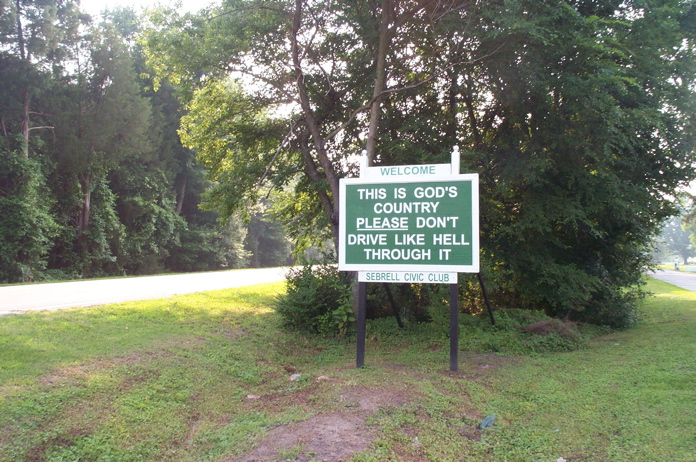The photograph depicts an outdoor scene centered around a distinctive sign with a mix of green and white backgrounds. The sign features the headline "Welcome. This is God's Country. Please Don't Drive Like Hell Through It." The word “please” is underlined for emphasis, all written in capital letters. The top of the sign includes a small white banner reading "Welcome," and the bottom displays another white banner with "Sebrell Civic Club" in green text. The sign is supported by two brown wooden poles and stands prominently in a grass and dirt patch, flanked by greenery and a large, fluffy green tree directly behind it. This tree is surrounded by additional trees lining both sides of what appear to be a rural road with paved surfaces and some areas of just dirt. The setting is reminiscent of a tranquil municipal-maintained boulevard with roadways running on either side, bordered by forested areas in the background.